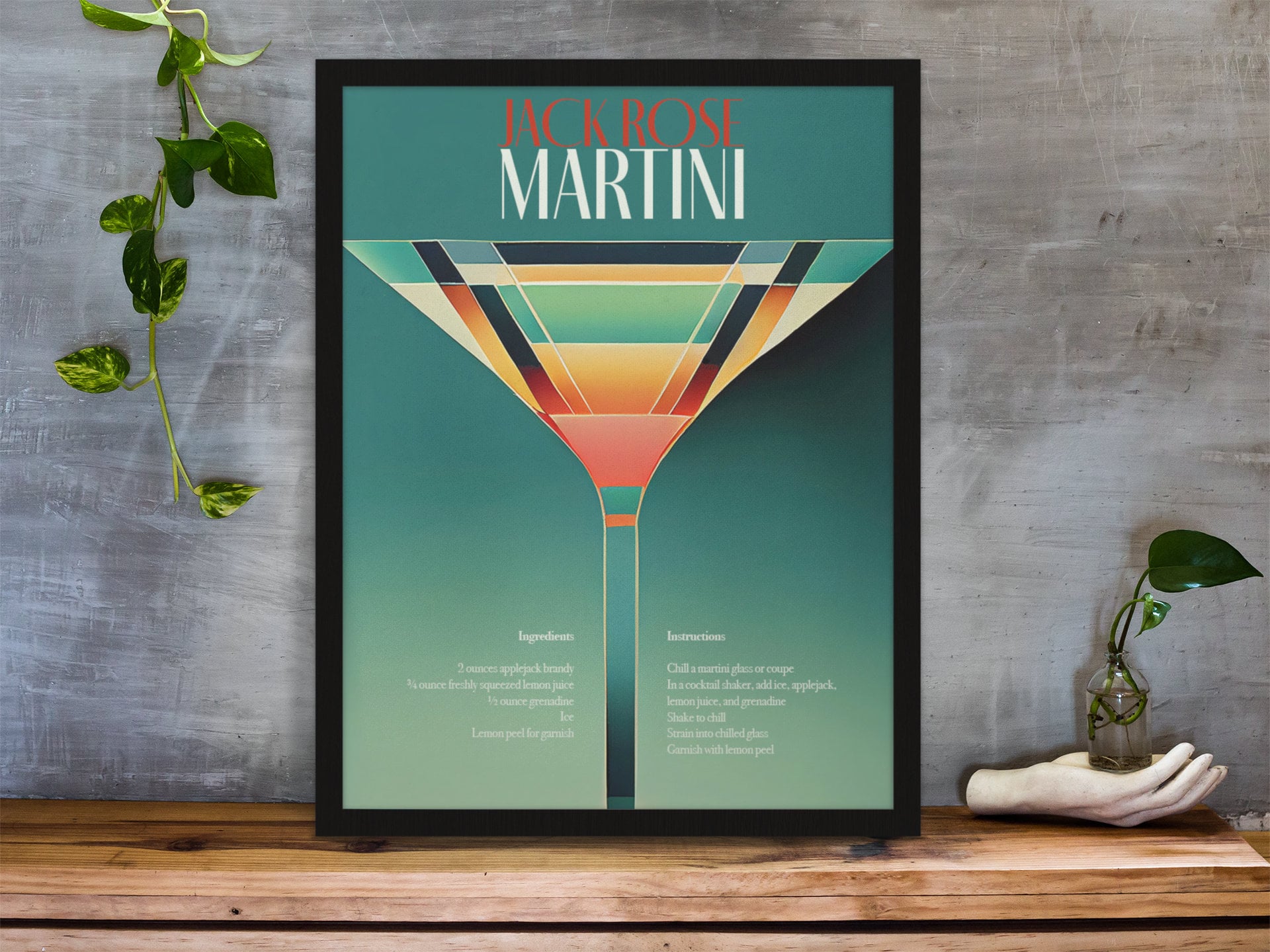The image depicts a framed print of a martini recipe labeled "Jack Rose," prominently displayed in bold red letters at the top, followed by "martini" in white lettering beneath it. The art piece features a modern pop art rendition of a martini glass, rendered through a combination of white lines and various geometric shapes in vibrant colors—reds, yellows, oranges, greens, and blues—creating a visually striking silhouette. This abstract martini glass is clipped off at the bottom and is divided into a colorful patchwork. The background of the print provides a list of ingredients on the left side and a set of instructions on the right.

The framed artwork, encased in a simple black frame, is leaning against a grey, concrete-like wall with subtle white streaks. The frame rests on a light tan wooden table, characterized by visible black knots in the wood grain. Adjacent to the framed print, to the right, stands a white statue of a human hand holding a small glass container with liquid and a plant featuring round, pointy green leaves. In the upper left corner of the image, a small portion of a house plant intrudes, adding a touch of nature to the backdrop. The detailed list of ingredients includes two ounces of Apple Jack Brandy, three-fourths of an ounce of freshly squeezed lemon juice, one half-ounce of grenadine, ice, and a lemon peel for garnish, all concisely laid out with corresponding instructions underneath. The overall image combines elements of artistry, design, and practicality, encapsulating the essence of the Jack Rose martini in a visually appealing setup.